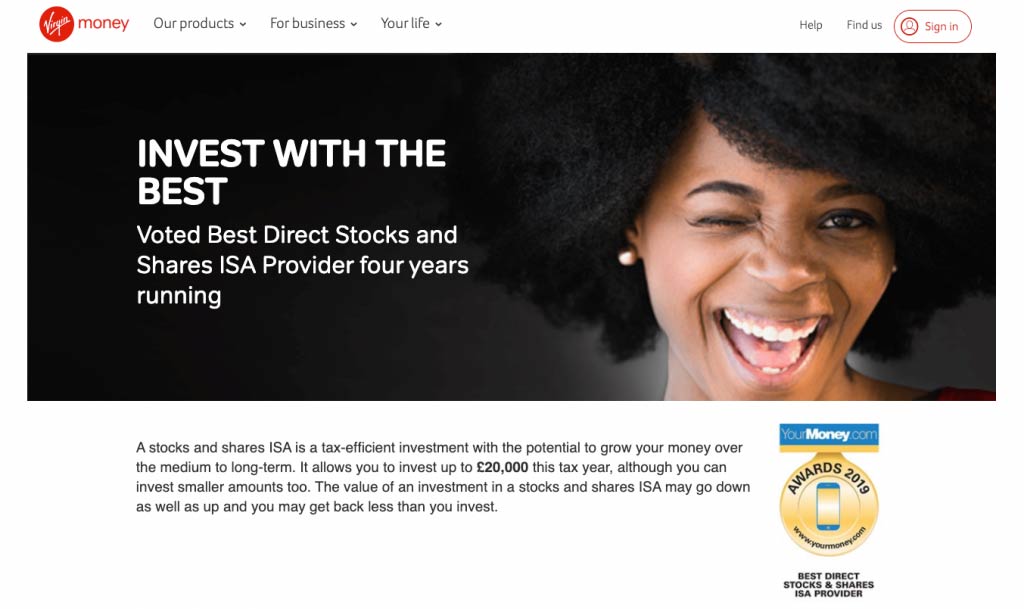Here is a detailed and clean caption for the screenshot image:

The image features a solid white background with text and a long horizontal photograph inside a rectangular box. The left side of the rectangular box has a black background with white text reading, "Invest with the best. Voted best direct stocks and shares ISA provider four years running." On the right side of the box is a photo of a young Black woman with curly black hair, winking and smiling broadly. Positioned in the upper left corner of the image is the Virgin Money logo, which consists of the word "Virgin" inside a red circle, and to its right are the words "money" in gray text. Above and to the right of the logo, gray text reads from left to right: "Our products," "For business," "Your life," "Help," "Find us," and "Sign in." Below the rectangular box at the bottom of the screen, there is additional explanatory text stating, "A stocks and shares ISA is a tax efficient investment with the potential to grow your money over the medium to long term."